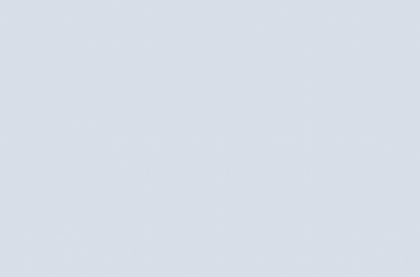The image depicts a simple, unadorned canvas of solid grey color. It lacks any discernible objects, text, numbers, or background elements. The entire rectangular frame is uniformly covered in this monochromatic shade, presenting an uninterrupted expanse of plain grey. There are no intricate details or stylistic features to be observed; just an empty, featureless grey surface spanning the entire image.